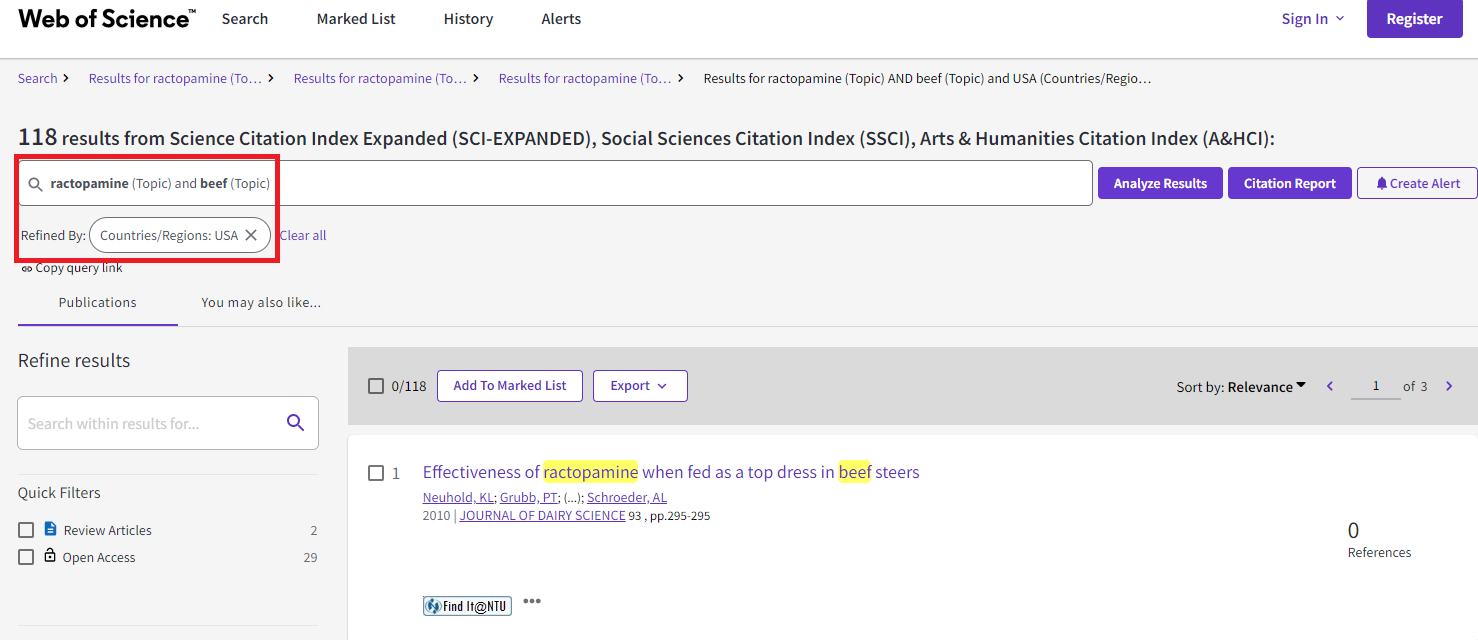This image captures a screenshot of a computer screen displaying the Web of Science web page. At the top of the page, there is a menu bar with options labeled "Search," "Marked List," "History," and "Alerts." The content below reveals that there are 118 search results retrieved from multiple indices: the Science Citation Index Expanded (SCI-Expanded), the Social Sciences Citation Index (SSCI), and the Arts and Humanities Citation Index (A&HCI).

Toward the left side of the page, within the section highlighting the 118 results, a hand-drawn rectangle emphasizes the term "ractopamine," which appears twice, both times mentioned under the search topics related to "beef." Additionally, the refinement options indicate the geographical focus "USA," with an "X" next to it, suggesting a filter applied to the search results.

Further scrutiny reveals a purple-colored "Sign In" area at the top right corner of the page next to a matching "Register" button. Just below these, there is a prominent purple box featuring options to "Analyze Results" and view "Citation Reports." This annotation likely serves as an instructional tool, possibly intended to guide users on how to navigate and utilize specific functionalities of the Web of Science platform.